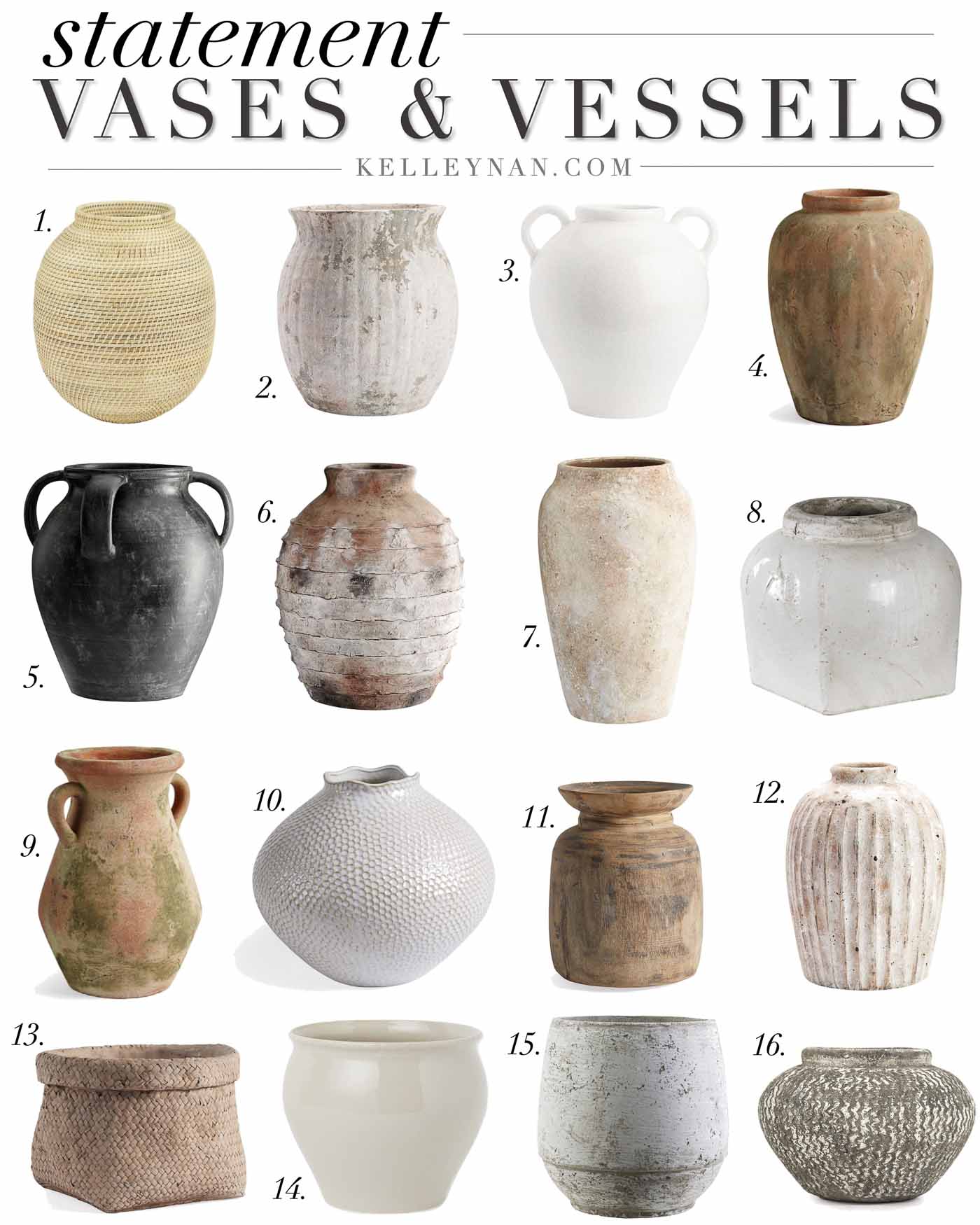This image, likely from a website named kellynan.com, showcases a grid of 16 distinct vases arranged in four rows and four columns against a white background. The top of the image reads "statement" in lowercase letters, followed by "VASES AND VESSELS" in uppercase bold letters, with a line above "statement" and another below "VASES AND VESSELS," and the website name "kellynan.com" written underneath. 

Each vase is numbered from 1 to 16, starting from the top left and ending at the bottom right. Vase number 1 is a wide-based, light brown vase that narrows at the top. Vase number 2 is a ceramic white vase with grey areas, giving it a rustic, vintage look. Vase number 3 is completely white with two small handles at the top, while vase number 4 is a brown, ceramic vase with a hint of orange. Vase number 5 is black with three handles, and vase number 6 has a honeycomb texture, featuring a brownish white color. 

Vase number 7 is a tall vase predominantly white, with green and pale brown accents. Vase number 8 is white and resembles a cookie jar in shape. Vase number 9 is a very rustic, old clay-looking vase with a brown and little bit of green color, and vase number 10 is another all-white vase with lots of texture. Vases 11 through 16 include a variety of designs, with vase number 13 shaped like a square bucket in light brown, and vase number 16 being a shorter gray and white vase with a wider middle than its top and bottom.